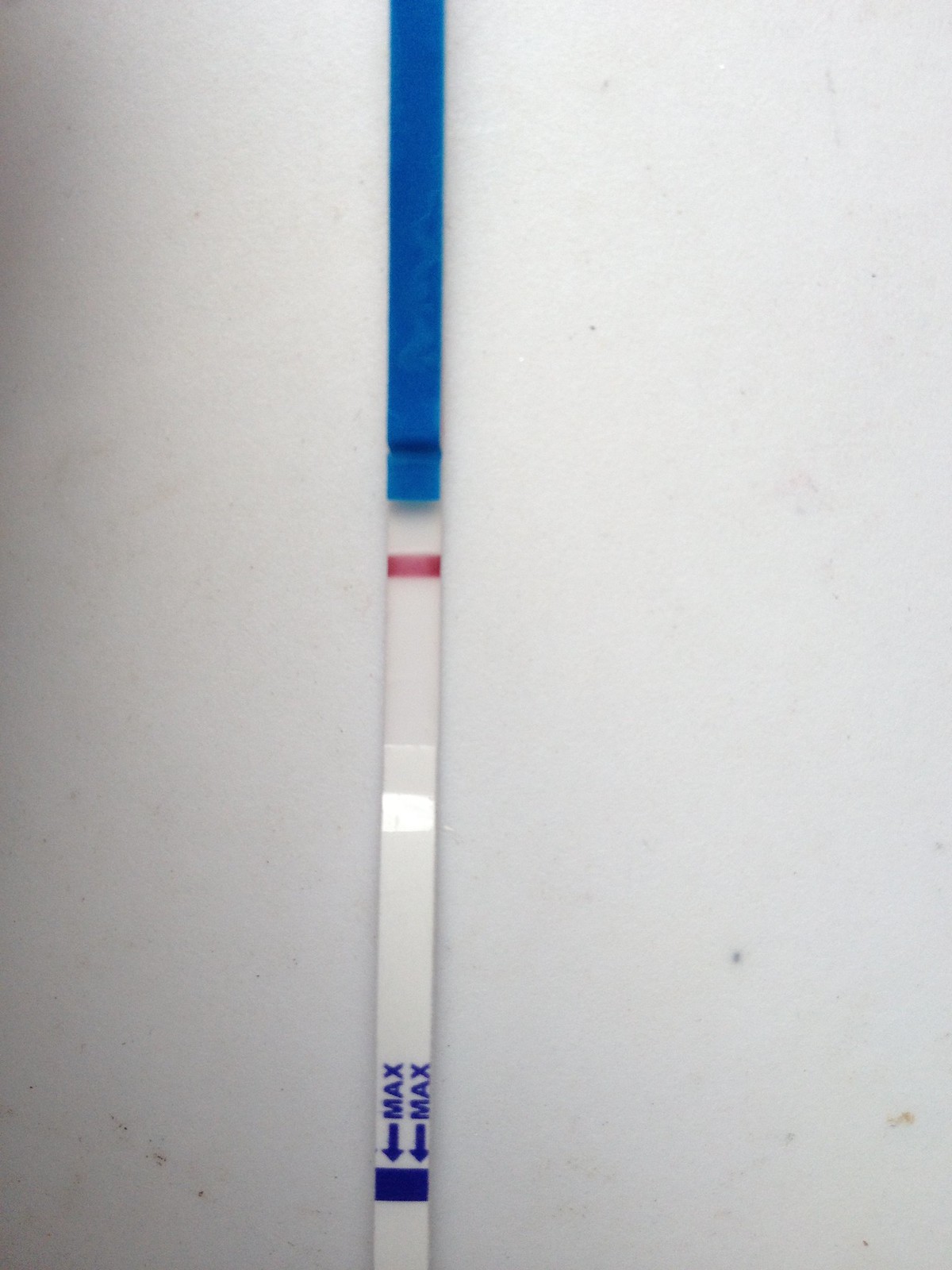A close-up photo captures an enigmatic object in portrait orientation, predominantly rectangular in shape but partially cut off at both the top and bottom edges. The backdrop is a white surface, marked with subtle dirt spots and shadowing in the corners, lending it a slightly darker and stained appearance.

The object features a dark blue section in its upper third, transitioning abruptly to a predominantly white color. About halfway down, a thin red stripe punctuates this transition, followed by a secondary, narrower blue stripe near the base, adjacent to some small text. The top blue portion, while roughly rectangular, narrows subtly towards its junction with the white area below. Beneath this junction point, in the white section, there is a small red stripe that disrupts the continuity. 

Further down, the white section dips inwards, creating a slight indentation with a reflective sheen. Near the bottom edge, two black arrows flank the printed word "MAX," pointing left and right towards the lowest blue stripe. This detailed configuration suggests that the object is likely a dipstick or fluid-level indicator, meant for gauging maximum fill levels.